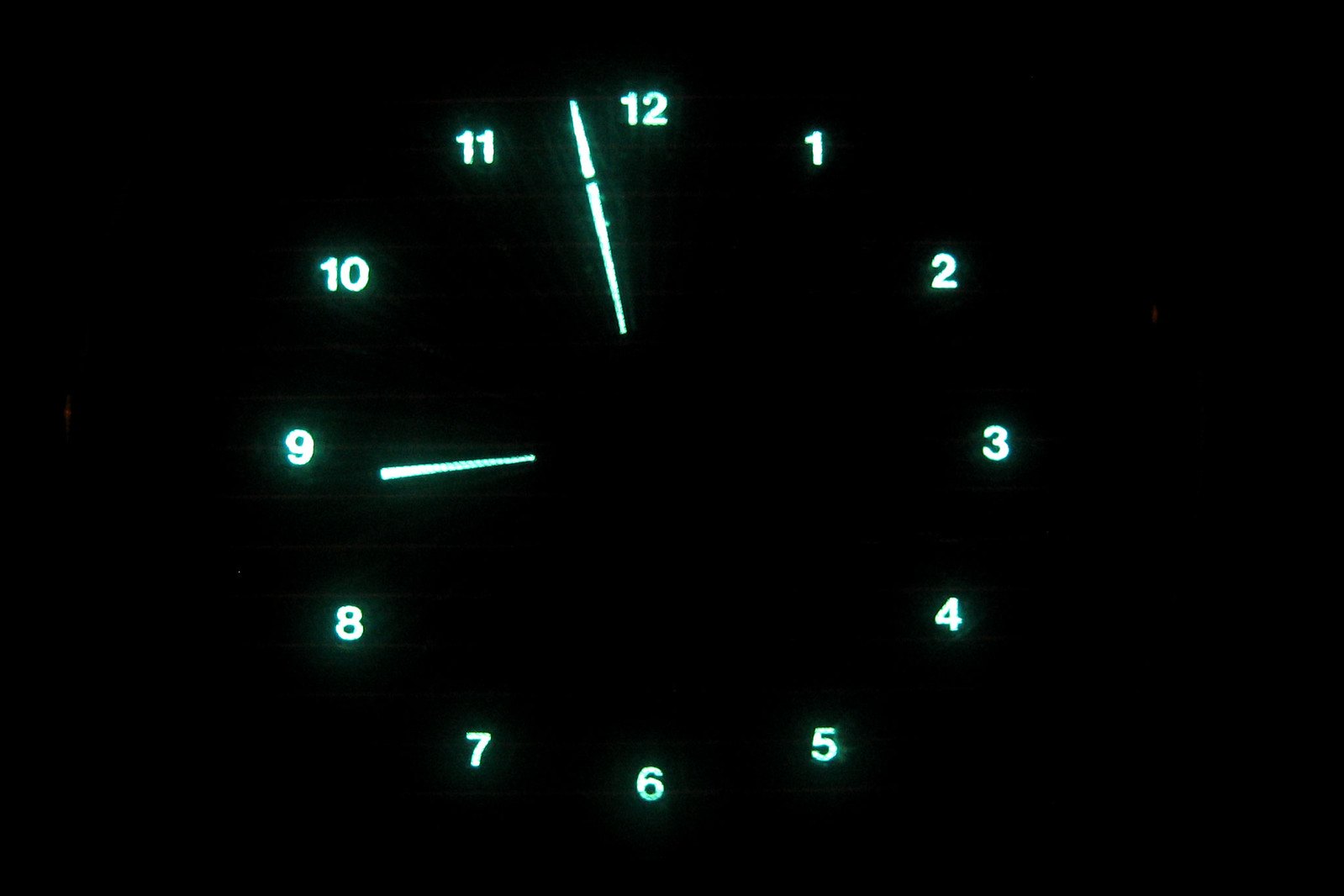In the image, a minimalist clock face is set against a black background. The clock displays a simple and clean design without any additional markings such as dashes or ticks. Luminous green LED numbers, ranging from one to twelve, are arranged in a circular fashion around the clock's periphery. The hour hand is positioned closer to the 9 o'clock mark, while the minute hand is midway between the 11 and 12, suggesting a time close to 8:55. The clock is illuminated in the dark, emphasizing the vibrant green LED numbers against the stark black backdrop, providing a modern and somewhat futuristic aesthetic.